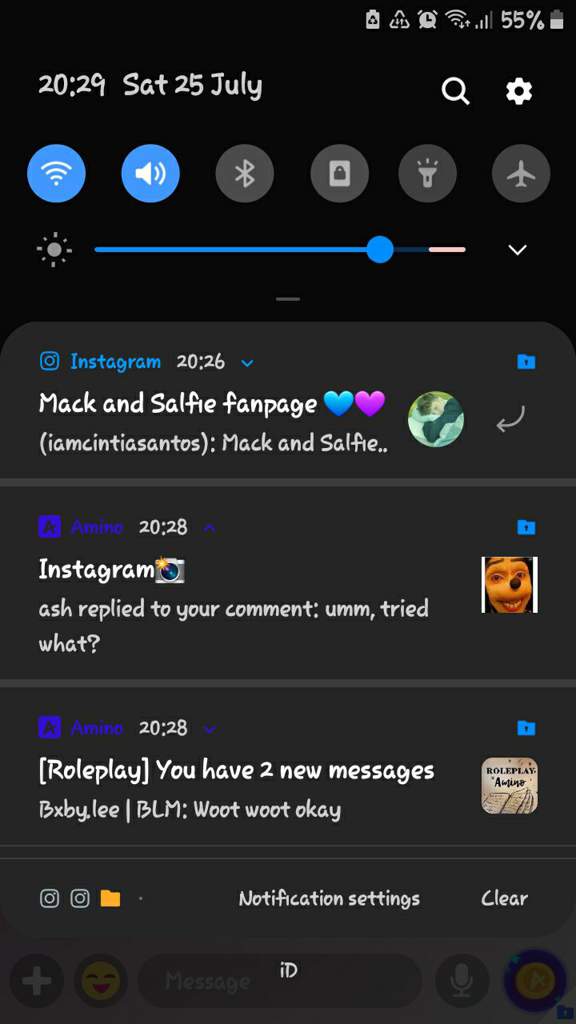The image features a complex and densely packed black background screen teeming with various icons and notifications. At the top, the battery level is displayed at 55%, and the date reads Saturday, 25th of July, 2029. 

Among the prominent elements, there is a magnifying glass icon for search and a settings icon. Additionally, there is a blue circle with soundwave lines indicating audio controls. Adjacent to it, several gray circles represent different functions: one with a bow, another with a lock, one featuring a light bulb, and another with an airplane icon, presumably for airplane mode.

A blue line extends with a round blue dot at its end, accompanied by a downwards arrow. 

Below these, there is a black box with a smaller blue box inside displaying the text, "Instagram 2026," followed by the label "Mac and Selfie fan page." This section includes a blue and a pink heart, the words "Mac and Selfie," and a black and white circular profile picture, highlighted by a pink descending arrow.

To the right, there is another blue box containing text and an arrow, leading to a section where "Amino" or "Amine" along with "2028 Instagram" and a camera icon are displayed. A notification reads, "Ash replied to your comment: tried what." A whimsical character image sits at the right side.

Further, there is a blue box with a plus sign at the top, suggesting an add function, followed by another segment indicating "Amine," detailing a role-play scenario and mentioning "you have two new messages" with the text "woot woot okay."

Towards the bottom, there's a notification box encapsulating text, another blue box with a plus sign for additional options, and an arrangement of icons: a square within a square, a camera-like icon, a brown file, notification settings, and a clear button. The ID section at the center highlights a round plus sign, a smiley face, a microphone, and what appears to be a gold coin icon.

Overall, the image portrays a bustling interface rife with social media activity, direct messages, and system notifications.